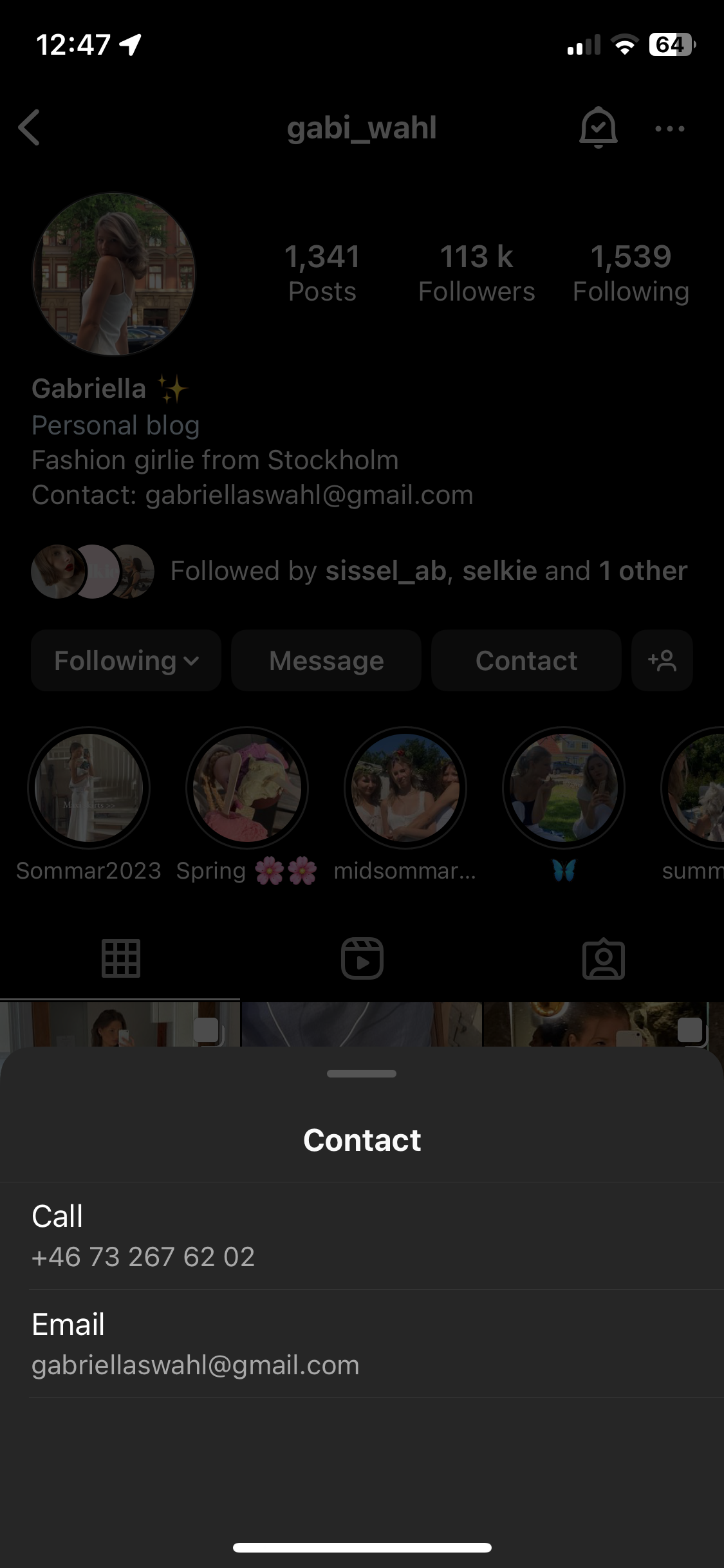Sure, here is a cleaner and more detailed Instagram profile caption:

---

This image showcases an Instagram profile with an open contact menu at the bottom of the screen. The background of the contact menu is black, and the white text reads "Contact." It provides a phone number, +46 732 676 202, and an email address, gabriella.swahil@gmail.com.

At the top of the image, part of the user's Instagram profile is visible. The user is Gabriella Wahil, with the handle @gabi_wahil. Gabriella has made 1,241 posts and has 10K followers and 1,539 followings. These details are positioned slightly to the right. On the left side of this section is the profile icon showing a woman in a white dress.

Below the profile icon, the name "Gabriella" is displayed, followed by a description, "Fashion blogger from Stockholm. Contact: gabriella.swahil@gmail.com." Additionally, it mentions that the profile is followed by users ccl_ap, silky, and one other.

At the bottom of the profile, there are options labeled "Following," "Message," "Contact," and "Add Friend." Just below these options, highlights of stories posted by the user are available, displaying the following titles from left to right: "Summer 2023," "Spring," "Midsummer," and an icon of a blue butterfly. 

The bottom part of the image lists the highlights as "Videos," "Private Videos," and "Contacts."

---

This refined caption provides a comprehensive description of the various elements present in the Instagram profile screenshot.